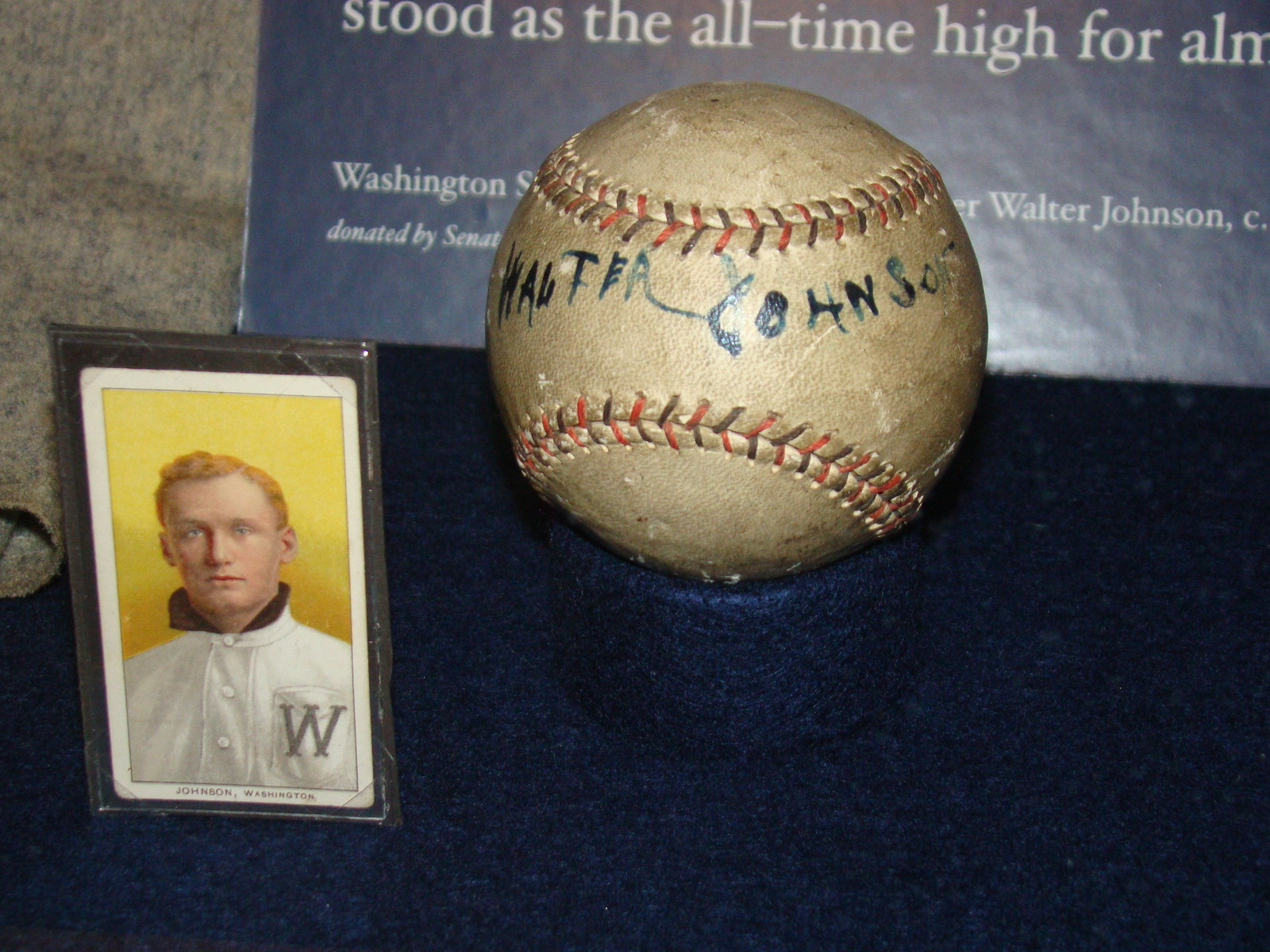The image showcases a vintage, weathered baseball with red and gray stitching, showing significant aging as the leather has turned brown. The baseball, marked with the signature "Walter Johnson," sits atop a round, black platform, which is set on a deep navy blue, velvety base. In front of the baseball is an old baseball card featuring a light-skinned man with short, wavy blonde hair, wearing a white baseball uniform with a black collar and a 'W' on his chest. The card text reads "Johnson, Washington." Behind the display is a blue board with white text, likely providing additional information about Walter Johnson. The entire setup resembles a museum exhibit, highlighting the historical significance of the baseball and its legendary player.